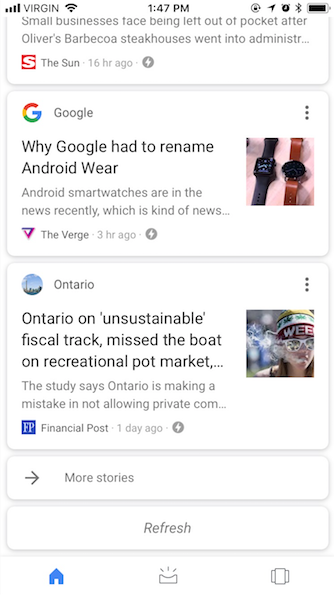This is a detailed screenshot from a mobile phone. The background is white, particularly in the upper left corner, where various status icons are visible. From left to right, there is a mobile signal icon accompanied by the text "Virgin" in black font, followed by a Wi-Fi icon with the time "1:47 p.m." displayed next to it. Further along, there's a series of icons: a lock, location sharing, alarm clock, Bluetooth, and battery.

Moving down, a small white rectangle with gray font contains the snippet: "Small businesses face being left out of pocket after Oliver's Barbacoa steakhouses went into administrate...". Adjacent to this text is a red square with a white "S" indicating it is from "The Sun" and marked as being published 16 hours ago. Nearby, a gray circle encloses a Thunderbolt icon.

Lower on the screen is another white rectangle. In its top left corner, there is a rainbow "G" icon next to the word "Google" in gray font. Below this, in black font, it reads "Why Google had to rename Android where Android smartwatches are in the news recently which is kind of news...". This article is from "The Verge," published three hours ago, and another gray circle with a white Thunderbolt icon accompanies it.

The final white rectangle at the bottom left corner features a blue circle icon with the text "Ontario" next to it.